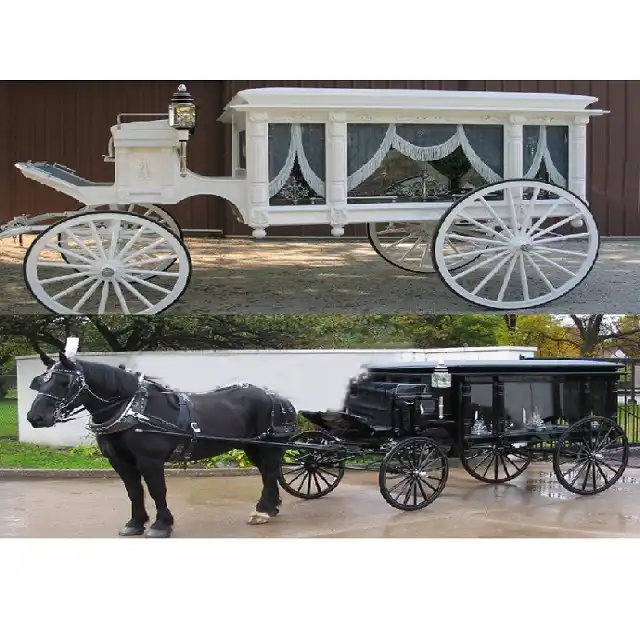In this detailed image, there are two distinct panels, each showcasing a different horse-drawn funeral carriage in an outdoor setting. The top panel features a white carriage with a detailed design that includes black drapes inside adorned with white tassels, large white-spoked wheels with black rims, and a lantern mounted at the front. The white carriage is situated near a barn and a wooden fence, resting on either pavement or dirt, and is notably devoid of any horses. The bottom panel presents a contrasting black carriage that appears to be a different but similar model to the white one, characterized by a lower top and an overall glossy finish, suggesting a wet cement surface. This black carriage is equipped with a black coffin and harnessed to a black horse, implying it's ready for a procession. Both carriages are intricately designed to serve as hearses, but the black carriage is actively engaged in its purpose, unlike the stationary white carriage.